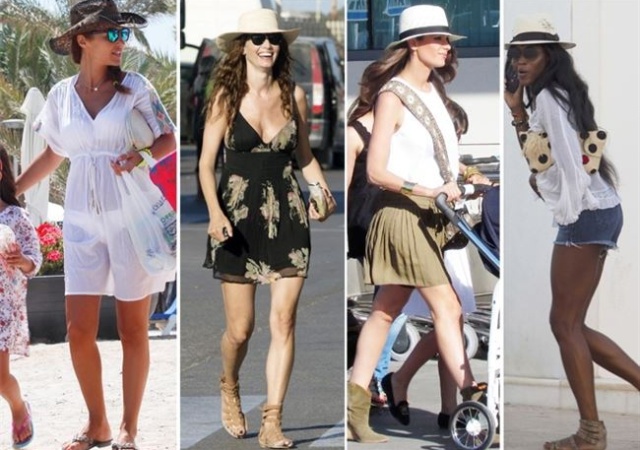In this image, four stylish women are captured walking outdoors, all flashing bright smiles. Two of the women are elegantly dressed in flowing dresses, while another wears a chic ensemble of a skirt paired with a short white top. The fourth woman showcases a more casual look, donning short denim shorts and a sheer white blouse. Positioned side by side from left to right, three of the women sport fashionable sunglasses, adding to their glamorous appearance, while the fourth goes without. All of them are adorned with trendy cowboy-style hats, effortlessly blending classic Western flair with modern fashion. Their relaxed demeanor and coordinated outfits suggest a fun outing or a casual stroll under the sun.